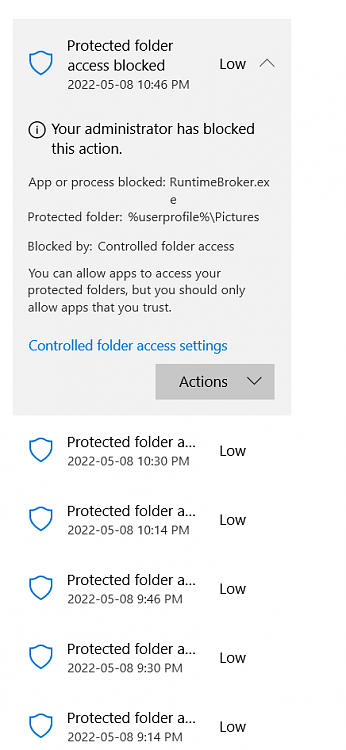The image showcases a screenshot from a mobile phone attempting to access a specific directory. It prominently features a gray notification box at the top, containing a blue-outlined shield icon with the text "Protected folder, access blocked" written in black. The notification includes a timestamp: May 8th, 2022, at 10:46 p.m. To the right of this message is a designation reading "Low" with an upward-facing caret (or arrow) beside it, hinting at additional information available upon interaction.

Beneath the main notification, text reads: "Your administrator has blocked this action," accompanied by an information icon—a black circle with a lowercase 'i' inside it. Further down, more details specify that the app or process is blocked, naming "RuntimeBroker.exe" as the responsible executable. The restricted access pertains to the user's profile folder, particularly the "user profile \pictures," protected by Controlled Folder Access. A note suggests that while apps can be granted permission to access these folders, only trusted apps should be allowed.

Additionally, there are options for adjusting settings, highlighted by the clickable blue text "Controlled Folder Access Settings." In the lower right corner of the grey box, there is another box labeled "Actions" with a downward pointing arrow, indicating possible actions the user can take.

Further down, the screenshot lists five prior access attempts to this protected folder, each marked with a blue-outlined shield icon. The logs indicate previous blocked access attempts on May 5th, 2022, at 10:30 p.m., 10:14 p.m., 9:46 p.m., 9:30 p.m., and 9:14 p.m., all flagged with a "Low" status. 

Conclusively, the image informs the user of multiple unsuccessful attempts to access a protected folder, with administrative restrictions and security measures actively preventing unauthorized access.